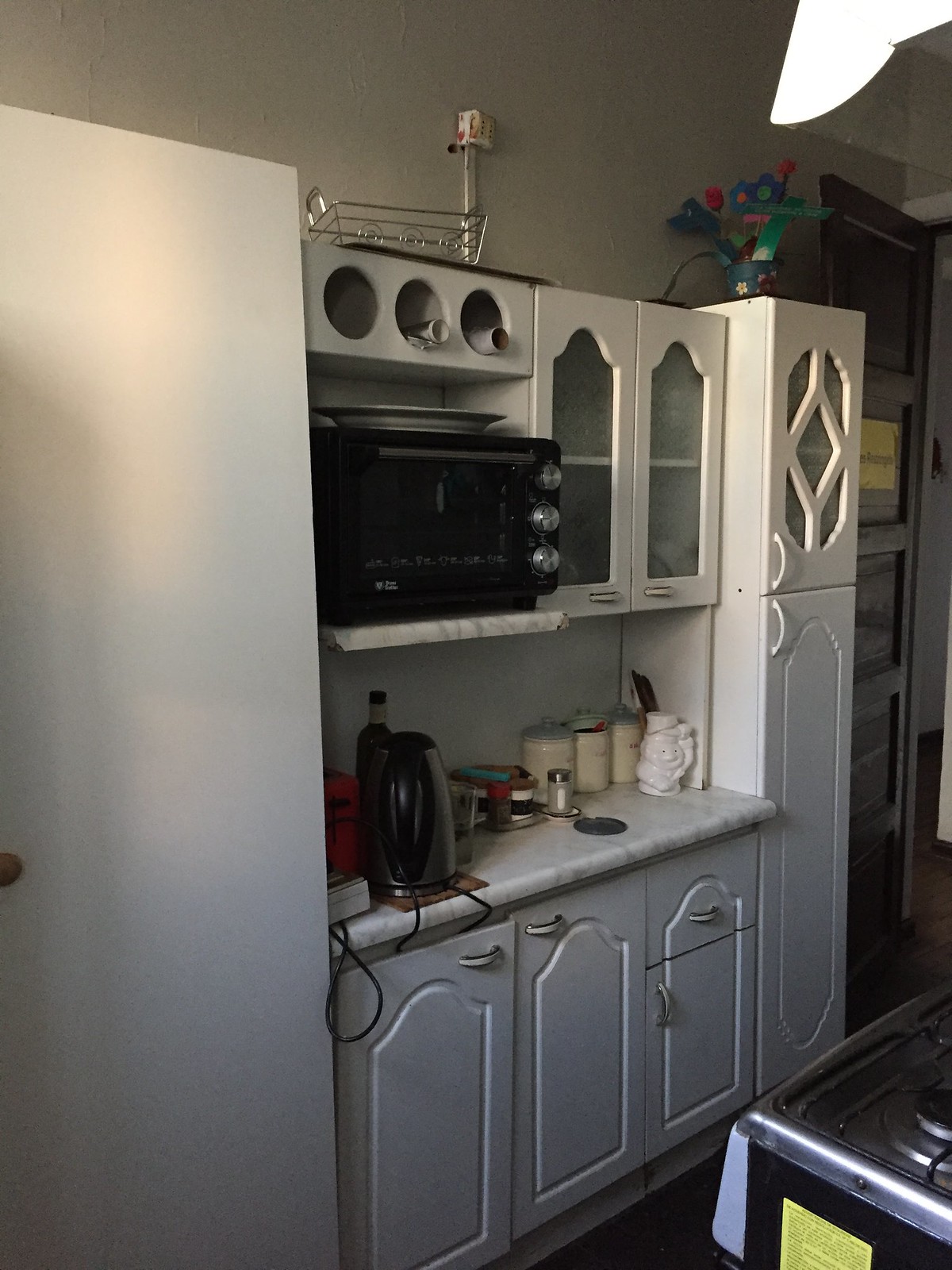This photograph captures a cozy, vintage kitchen inside someone's home, reflecting a design from several decades ago. The small galley-style space is characterized by white cabinetry, adorned with old-fashioned arches and embellished with designs. Two of these cabinets feature clear glass doors, ideal for displaying chinaware.

On one side of the kitchen, a gas stove peeks in from the lower right corner. The countertops are a white marble, hosting a range of kitchen essentials including sugar and flour canisters, salt and pepper shakers, and a coffee maker. In the back corner stands a wine bottle and a small container of salt.

A black microwave with three silver knobs is mounted on a shelf, above which are circular openings holding rolled-up items like posters or foil. There is also a black electric tea kettle and a colorful fake plant in a wire basket on the countertop. The tall cabinet to the right features a glass-paneled door at the top, while the leftmost cabinet has a glass door with clear windows.

Adding to the nostalgic charm, there’s a wooden door with a brown finish leading into the kitchen. Despite its compact size, the space is well-utilized and exudes a comfortable, lived-in feeling.